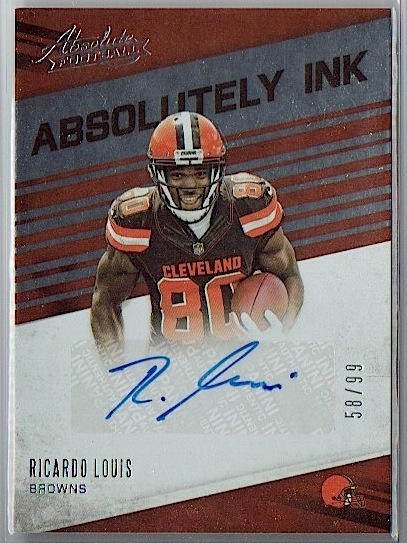This is an autographed football card from the brand Absolute, likely a Panini product. The card features a muscular football player, Ricardo Lewis of the Cleveland Browns, prominently in the center. He is wearing a brown jersey with orange letters and numbers that spell out Cleveland number 80, and he’s carrying a football in his left hand. The player's helmet is orange with distinctive brown and white stripes. The card has a colorful design with red and gray stripes running across the top, and a silver-stamped "Absolute Football" logo is located in the upper left corner. Just below the logo, the words "Absolutely Ink" are written in black. There is a sticker autograph from Ricardo Lewis placed inside a large white stripe at the bottom of the card. On the left side, the player’s name is clearly marked as Ricardo Lewis Browns. On the right side of the card, the text "58/99" indicates its serial number, with only 99 such cards produced, and this particular one is number 58. Below this, there is a small orange graphic of a Cleveland Browns helmet. The player is looking towards the viewer, enhancing the connection between the card and its audience.